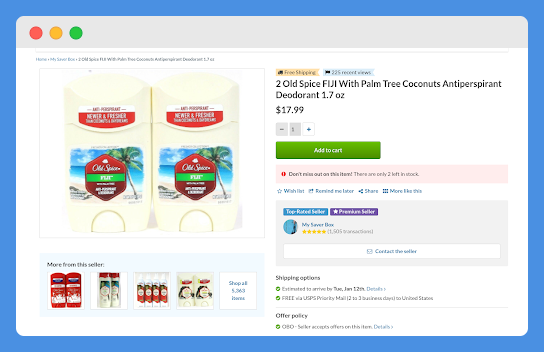The image features a product display with a blue border surrounding all four sides. Inside the blue border, a gray border is positioned at the top. Within this gray section, there are three colorful circles: one red, one orange, and one green. The primary focus of the image is two sticks of Old Spice deodorant, labeled "Newer and Fresher Old Spice Fiji." The deodorant sticks have a beach-themed label depicting palm trees, sand, and a clear sky.

To the right of the deodorants, the text advertises "Free Shipping" for the Old Spice Fiji antiperspirant deodorant, with each 1.7-ounce stick priced at $17.99. Beneath this text, there are minus and plus buttons to adjust the quantity, with a number "1" displayed between them. Below these buttons, a prominent green "Add to Cart" button is visible. Further down, although slightly blurred, the text appears to offer options such as "Wish List," "Reserved for Later," "Shipping Option," and "Offer Policy."